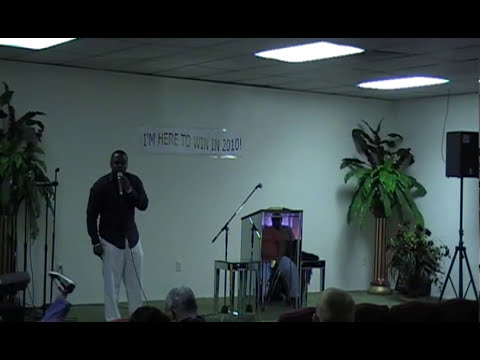In the image, a black man, dressed in a black shirt and white pants, is giving a speech on a stage. He is holding a microphone close to his face, and a cord trails from the microphone. The scene is slightly dim, with the image having an overcast hue of light black. The stage is flanked by tall, potted greenery, with large palm-like plants visible on both sides. Behind him, the white wall displays a banner that reads, "I'm here to win in 2010!" in bold print. The white ceiling above is lined with fluorescent panels providing overhead lighting. Additional elements include several microphone stands scattered across the stage, a set of speakers on a tripod to the right, and a grand piano positioned centrally. The area also contains an oddly-shaped podium, with a second man seated inside, and amp equipment. In the foreground, the tops of the heads of audience members can be seen, indicative of the event's attendance. There is a peculiar detail of a foot, or possibly a shoe on a hand, visible at the bottom left corner of the image. The setting suggests a formal gathering or motivational talk, potentially with a religious or educational context.